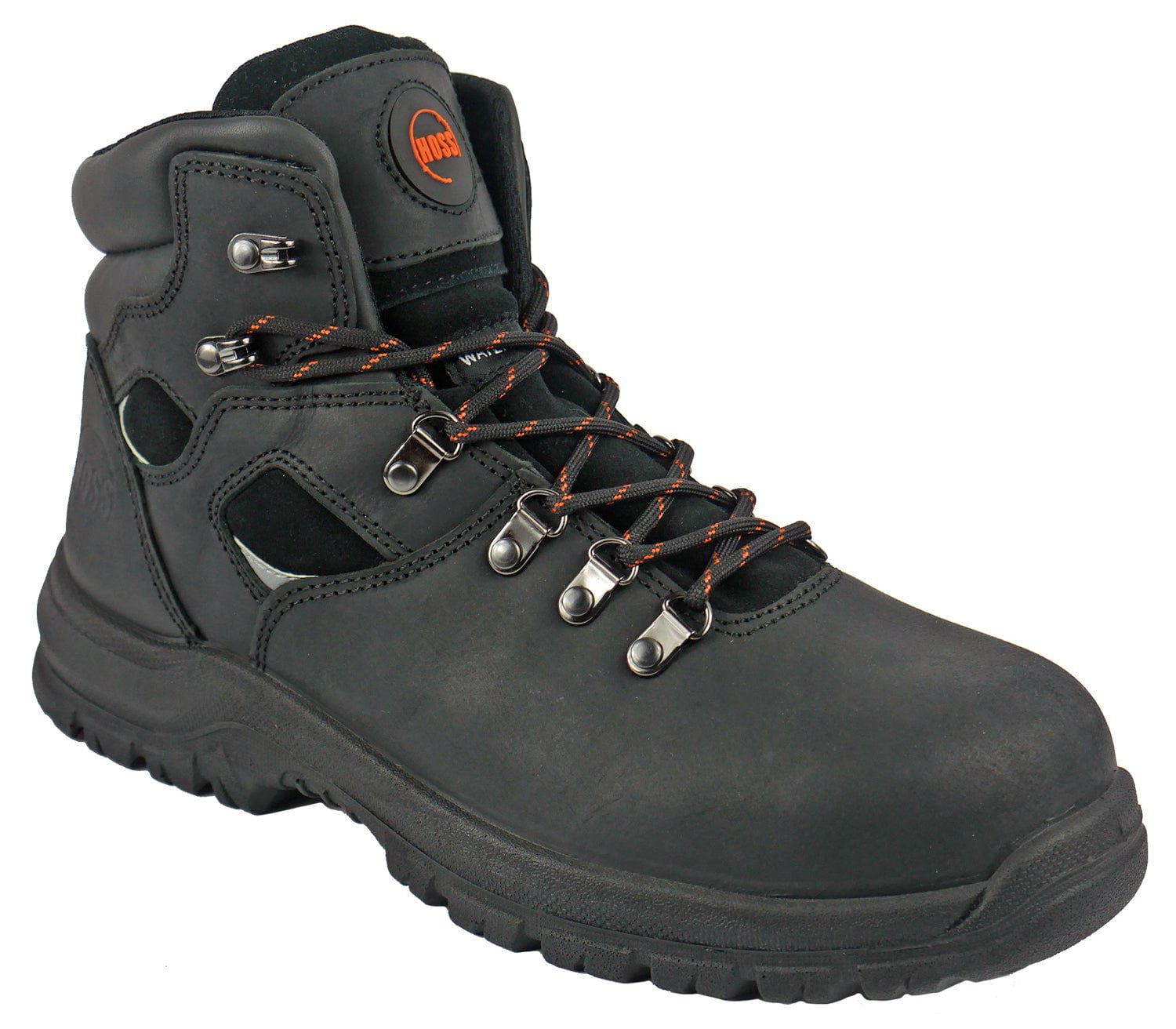This marketing-style close-up photograph showcases a high-top black boot, designed for heavy-duty work, positioned against a stark white background. The boot, which is facing right with the toe in the lower right corner and the heel near the middle left edge, features a sleek black faux leather upper and a robust rubber sole with deep tread suitable for extensive wear. The upper part of the boot is predominantly black, with a darker shade used for the interior elements such as the tongue and laces. The boot's tongue boasts a prominent red logo reading "Haas," punctuated by a circular design. Red dotted lines add a touch of personality to the black laces, which are threaded through metal eyelets. Notably, the laces are not completely fastened, with the topmost eyelet left unused. The tongue also includes a soft mesh section transitioning into the same leather material found throughout the boot. Intricate double stitching and heavily sewn leather binding reinforce the ankle area, ensuring durability and support. This entire composition hints at the boot’s suitability for rigorous environments, combining functionality with subtle design elements for a polished, sturdy appearance.